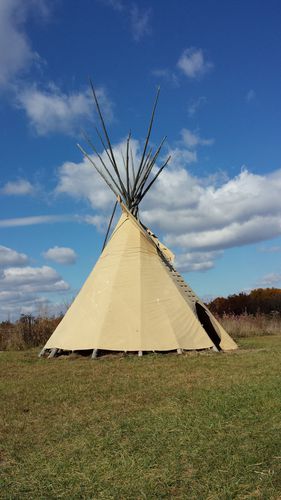The image depicts a traditional teepee, primarily tan and brown in color, although it appears to be made from cloth rather than authentic skin. The teepee is constructed with numerous long poles, which extend high above the conical structure, all tied together at the top to form the framework for the covering. The entrance flap of the teepee is visible on the right side of the image. It sits on a large expanse of green grass interspersed with some brown patches, surrounded by a backdrop of trees. The sky above is a bright blue adorned with puffy, white clouds, adding to the serene and picturesque setting. No signs of current habitation are evident, but its authentic construction suggests a respect for traditional methods.